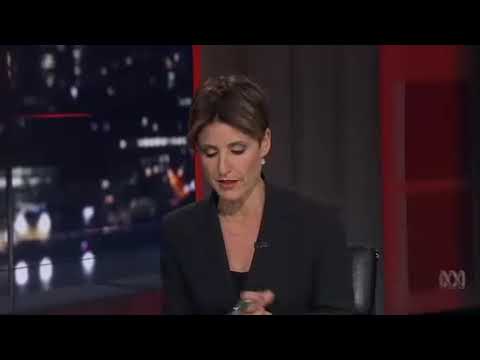The image is a still shot, possibly from a TV broadcast, showing a Caucasian woman with short brown hair, which is parted in the center and likely pulled back. She is seated in a black, conservative business suit with a simple lapel and a black shirt underneath, on a black chair. Her minimal makeup accentuates her red lips. The woman appears to be looking down at a desk, with glasses and possibly a green pen in her clasped hands. A microphone is attached to her lapel. The background features a nighttime cityscape with lit buildings on the left, a gray curtain or wall directly behind her, and red accent lighting on a white surface to the right. The image is letterboxed with thin black rectangles at the top and bottom, and in the lower right corner are the letters "XX" in parentheses.